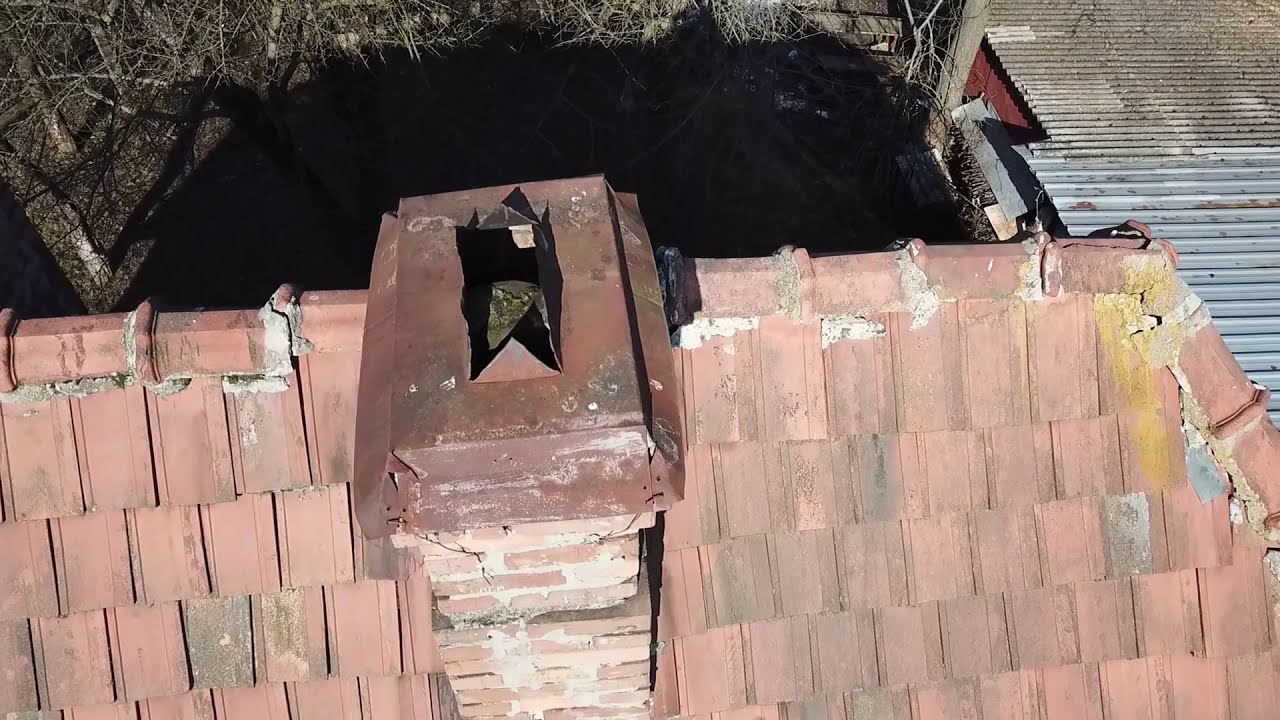The photograph captures a weathered rooftop with distinct red tiles in a state of disrepair, featuring numerous chips and an overall worn appearance. In the center of the roof stands a crooked brick chimney, constructed from red bricks bound by concrete. Atop the chimney sits a heavily rusted metal cap, which appears to have been cut open. To the far right, a structure with a corrugated metal roof is visible, its surface transitioning from silver to brown, possibly covered in leaves. Below the roof is a dark, murky body of water, bordered by sparse, leafless trees and vegetation. The surrounding area includes dirt, debris, and sticks, suggesting a neglected environment.